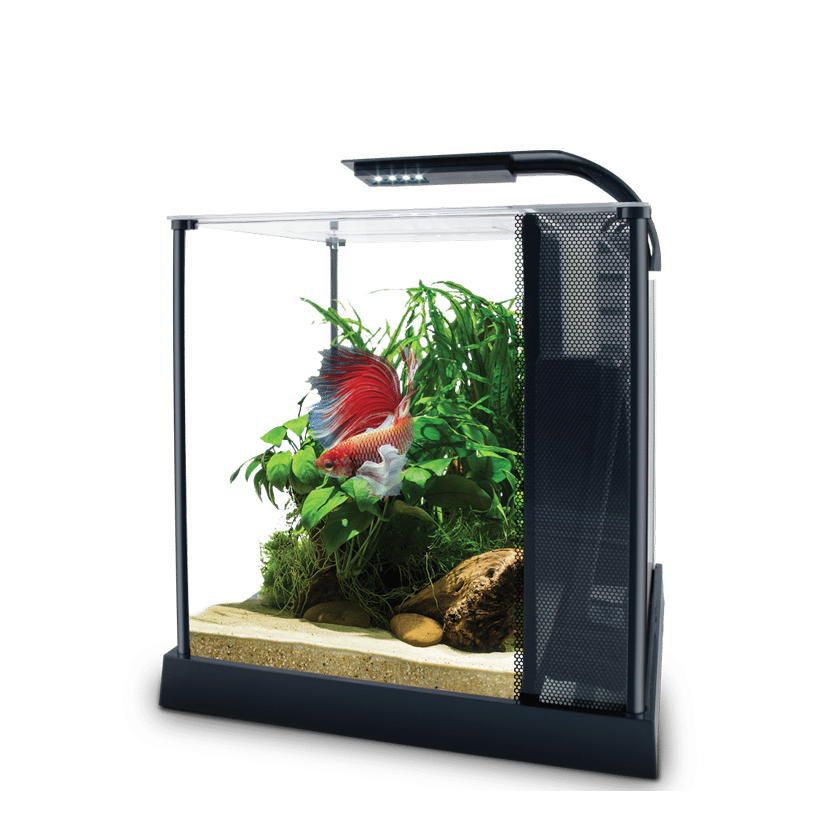The image depicts a detailed and intricate fish tank system that is both functional and aesthetically pleasing. The aquarium itself consists of a seamless glass box mounted on a sturdy black base. The base appears to be made from a durable material like plastic, metal, or possibly wood, and it features four dark, round beams at each corner that support the structure. Atop the aquarium is a sleek, dark-toned light fixture, which may include UV bulbs for additional sanitation.

Inside the tank, the scene is vibrant and lively. There is a layer of sand covering the tank's bottom, accented with an arrangement of stones and lush water plants that create a verdant underwater landscape. Towards the left side of the tank, a striking tropical fish with an elaborate and wide, red tail, accented with light teal hues, swims gracefully. Its tail fans out in a magnificent display, reminiscent of a peacock’s plume. The fish’s presence is complemented by the crystal-clear water, which allows an unobstructed view of the interior elements.

Additionally, on the right side of the tank, there is a noticeable black component that curves up and over, which likely serves as the filtration and circulation system, integral to maintaining the tank's pristine environment. The combination of these elements creates a harmonious and visually appealing aquatic habitat, perfect for showcasing the elegant beauty of the fish and plant life within.